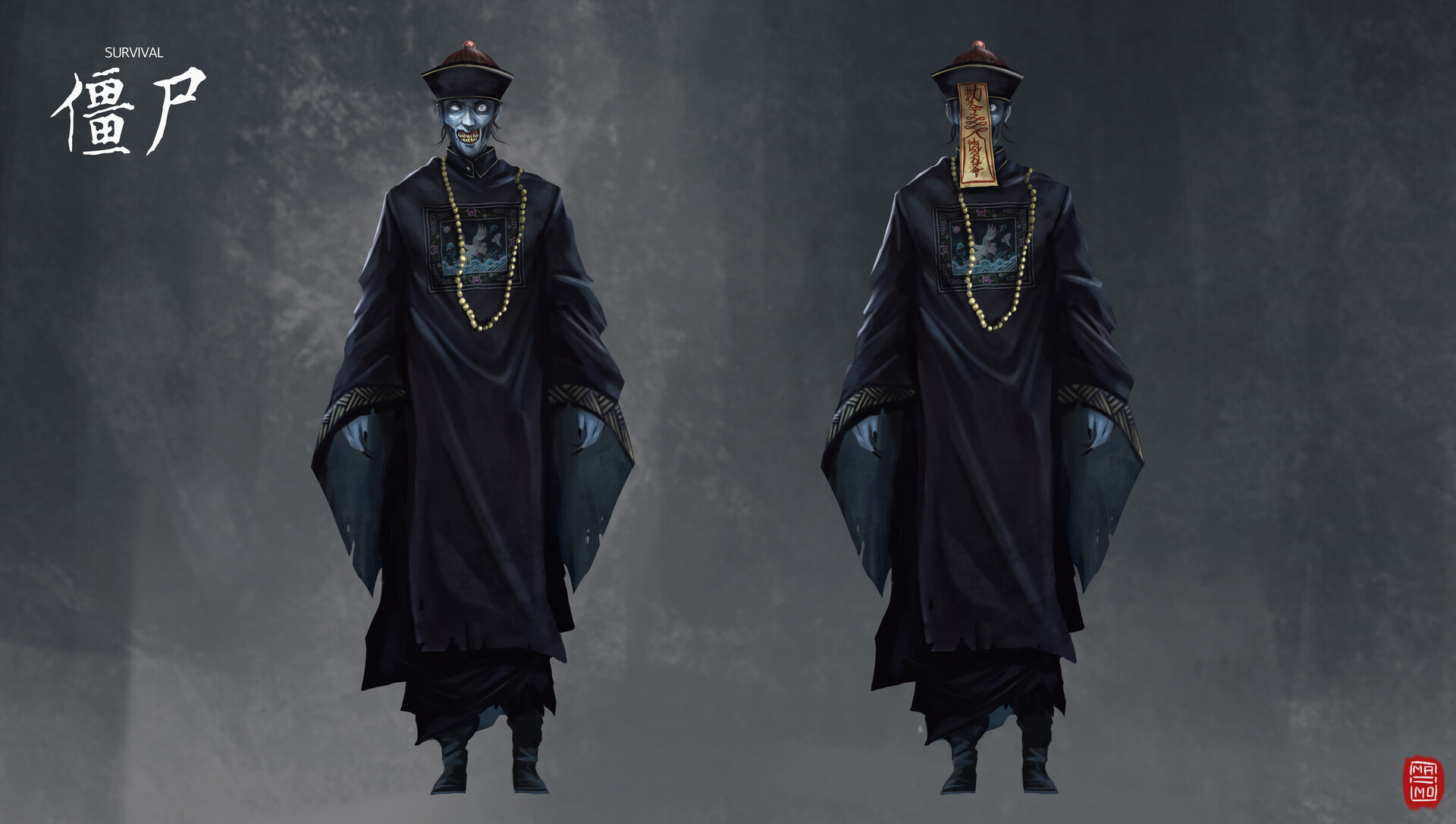The image appears to be an advertisement for a video game, featuring two distinct, gaunt, human-like characters with light blue skin standing side by side against a background of varying shades of gray, from charcoal to light gray. The character on the left has a skeleton face with glowing gray eyes, covered by a pointed hat and wearing a long, black, cloak-like dress with black boots. Its gray hands possess black, pointed fingernails. It accessorizes with a long necklace made of gold beads that hangs down to its waist. The character on the right dons similar attire but has a tan parchment banner over its face that extends to its neck, adorned with Chinese writing. The upper left corner of the image has the word "survival" followed by Chinese symbols, while the bottom right corner features a red label with the initials "M.A. M.D." Additionally, the background includes faintly visible ghostly trees and snowy ground, contributing to the eerie atmosphere.